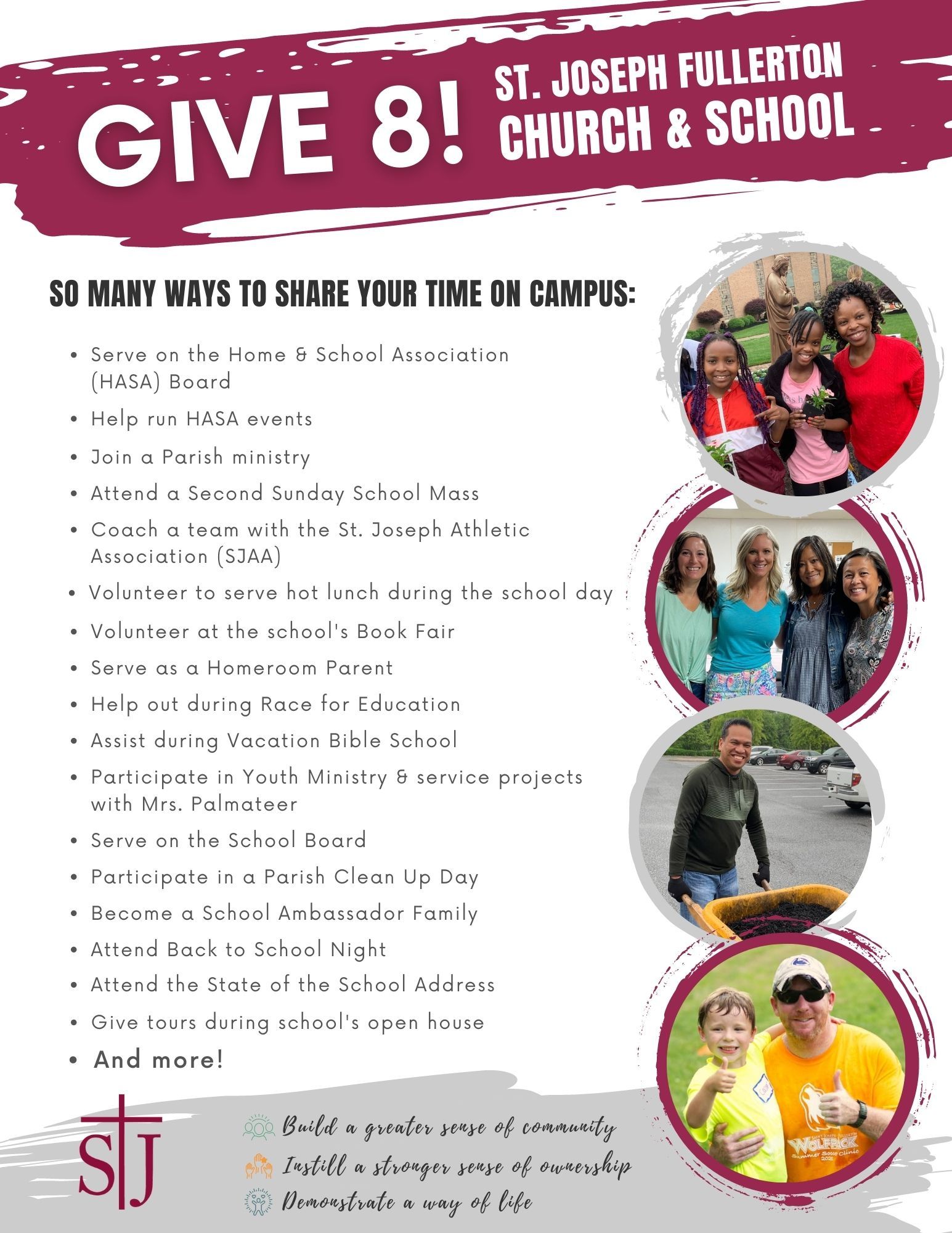The image showcases a white brochure with a magenta-colored brush stroke at the top featuring white text that reads, "Give Eight! St. Joseph Fullerton Church and School." Below the heading on the left side, there is a black-text bullet list titled "So many ways to share your time on campus." The detailed list suggests numerous volunteer opportunities, such as joining the parish ministry, helping with HASA events, serving hot lunch during school days, attending dress gift tours during school openings, and coaching a team with the St. Joseph Athletic Association (SJAA). On the right side of the brochure, there are four vertically stacked circular images. The first image shows three women smiling, the second features four women smiling, the third depicts a man smiling while carrying a wheelbarrow, and the fourth captures a father dressed in yellow, enjoying a sunny day. The bottom of the brochure displays the St. Joseph Fullerton logo, which consists of the letters "S" and "J" with a cross in the middle, and a tagline that reads, "Build a greater sense of community, instill a stronger sense of ownership, and demonstrate the way of life."